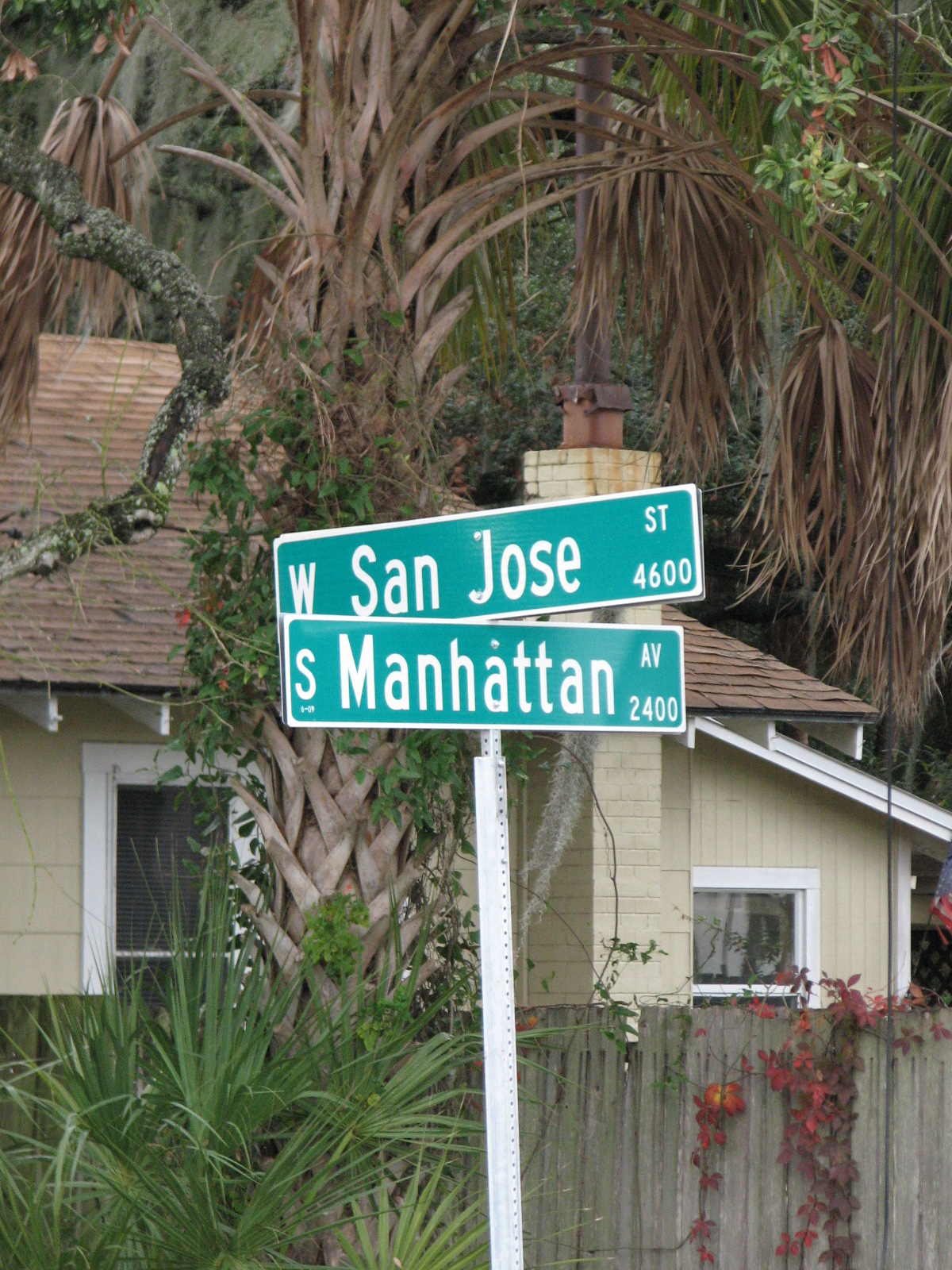In the photograph, we are looking at an intersection marked by a street sign. The sign comprises two green rectangular boards with white writing, mounted one above the other. The top sign indicates "West San Jose Avenue," running east-west, while the bottom sign points out "South Manhattan Avenue," extending north-south. Nestled in a residential neighborhood, the scene includes a beige-colored home accented with white trim and topped with a brown roof. The background is framed by an array of lush palm trees, their green fronds contrasting against the sky. Adding to the picturesque view is a privacy fence adorned with vibrant red flowers and climbing ivy. The green and brown hues of the foliage provide a rich, natural backdrop to the tranquil suburban setting.